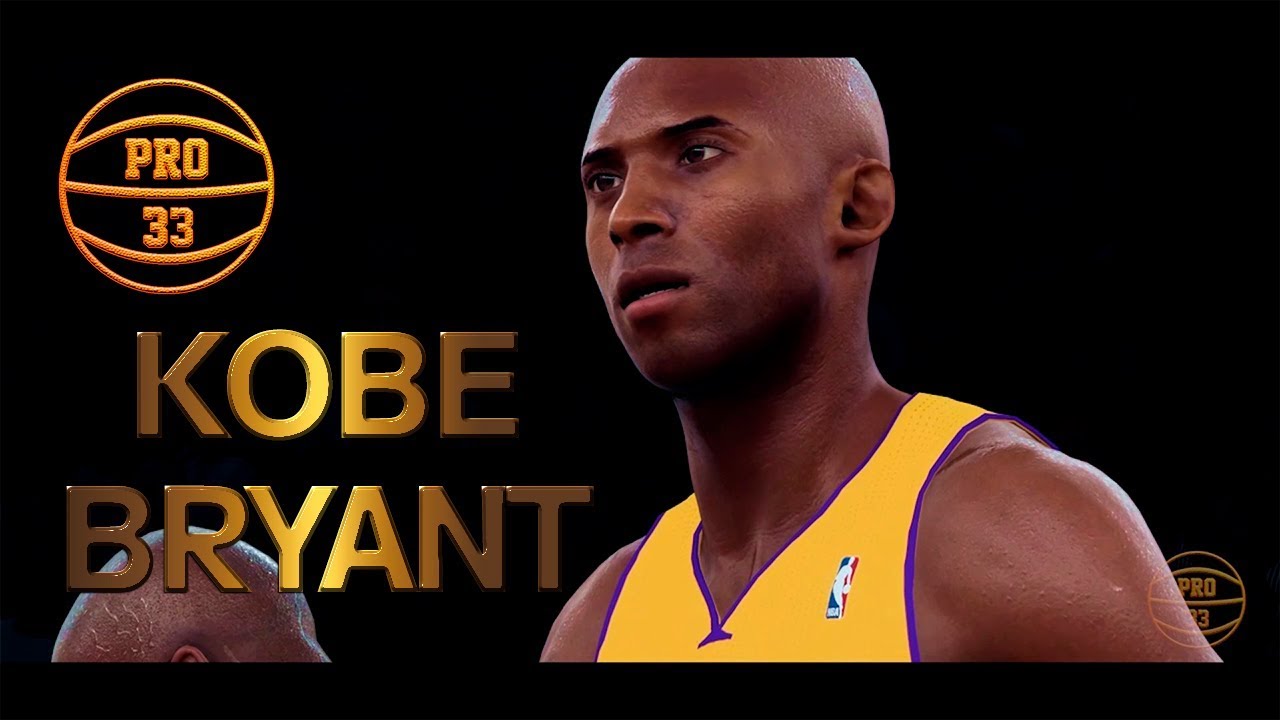This digital rendering showcases Kobe Bryant in a highly realistic and emotive depiction, likely from one of the 2K sports games. Kobe, an iconic figure in professional basketball, is prominently featured at the center. He stands fully visible, his expression marked by disbelief as he gazes intently at a point off-screen. Kobe's figure is rendered with incredible detail, from his bushy black eyebrows and clean-shaven face to the muscles on his shoulders. He is wearing a yellow jersey accented with purple lines and adorned with the iconic NBA logo—a white silhouette with a basketball overlaying a blue and red backdrop.

To the left side of the image, a digitally created golden yellow basketball is featured, emphasizing the 'PRO' label in bold gold and yellow lettering. Below the basketball, Kobe's name is displayed, with 'Kobe Bryant' partially illuminated and glowing through the letters 'O', 'B', 'Y', and 'A'. The letters 'B', 'E', 'N', and 'T'—as well as 'K' and 'BR' at the beginning—fade into a black-gold mixture, blending subtly with the background.

A second, less visible figure—of African-American descent—is partially rendered to Kobe's left. This individual is only shown from the back, capturing just the head and ear, their presence adding depth to the scene without diverting focus from Kobe. The background remains predominantly black, except for another basketball in the lower right-hand corner that mirrors the one described initially, featuring the same 'PRO' label and decorative elements. The overall composition highlights Kobe's impactful legacy while merging artistic elements with the realism of digital sports graphics.